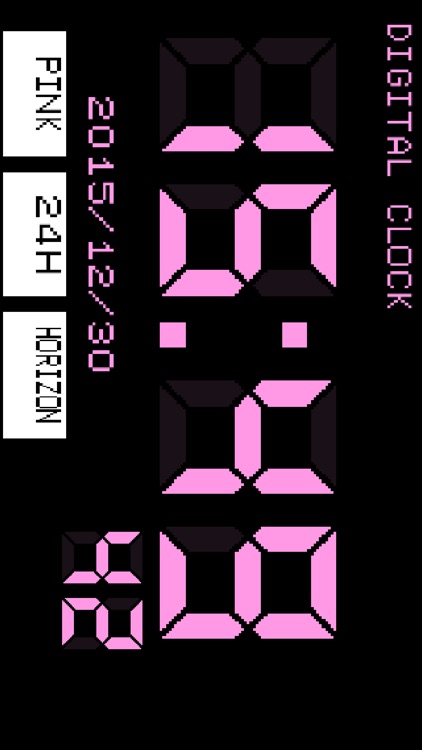The image depicts a sideways digital clock with a black background. The text is oriented from top to bottom, forming a vertical rectangle. On the right side, in pink text, it reads "digital clock." Dominating the center of the image is the time displayed in large, block-style pink numbers: "1549," with the number "42" below the "9." Directly beneath the "15," the date is shown as "2015/12/30." On the far left of the image, there are three white rectangular boxes with black text inside. The top box reads "pink," the middle box reads "24H," and the bottom box reads "horizon." All these elements are aligned vertically due to the orientation of the clock face.